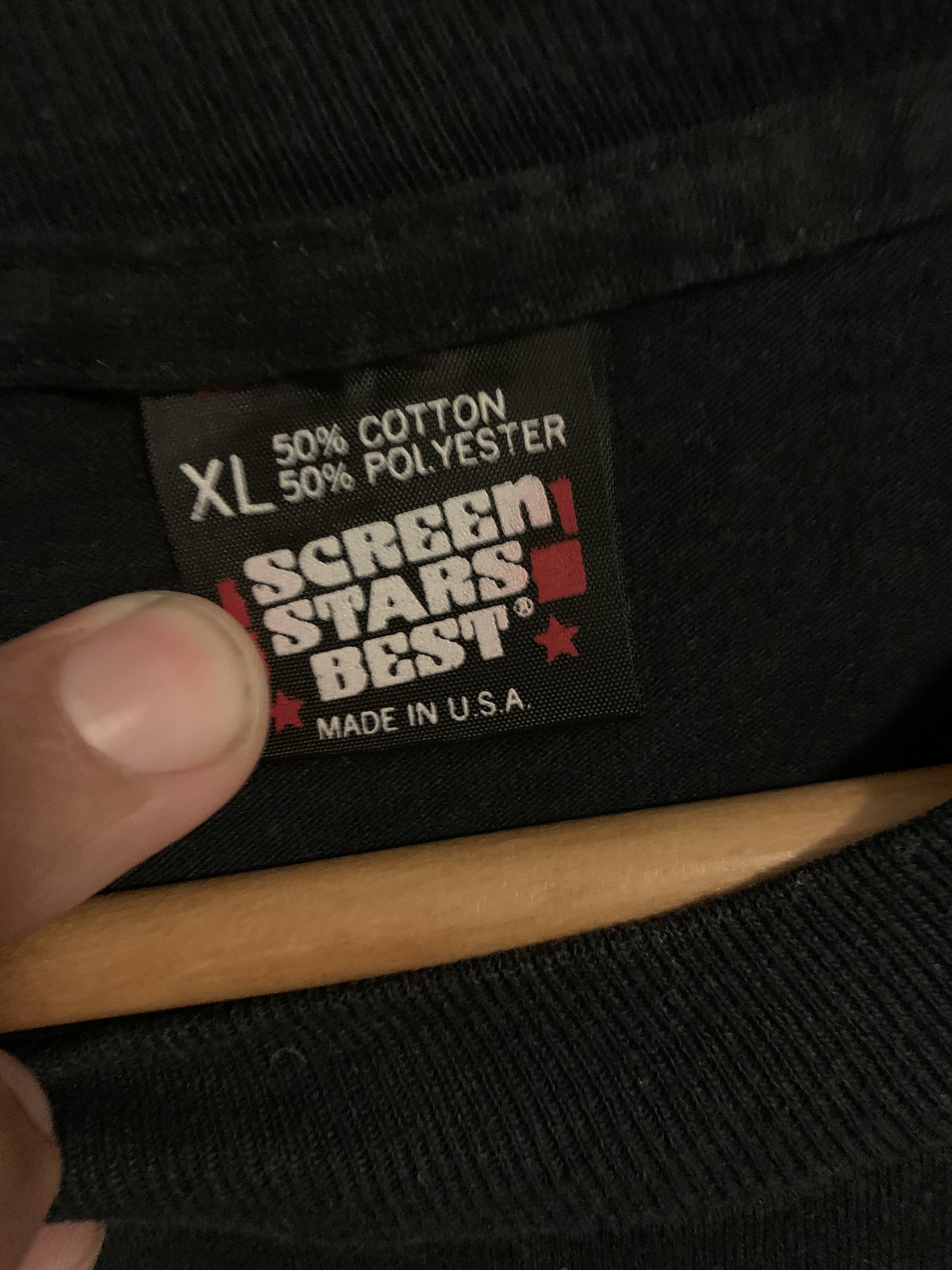This close-up image features a black garment, likely a t-shirt or sweater, highlighted by a detailed view of its tag located inside the collar. The black tag, adorned with white text, prominently displays "XL," indicating the size as extra-large. Below the size, it specifies the fabric composition as "50% cotton, 50% polyester," followed by "Screen Stars Best, Made in USA." The focal point of the picture is the tag, firmly held down by the thumb of an off-frame hand. Additionally, a wooden hanger is partially visible, extending through the collar.